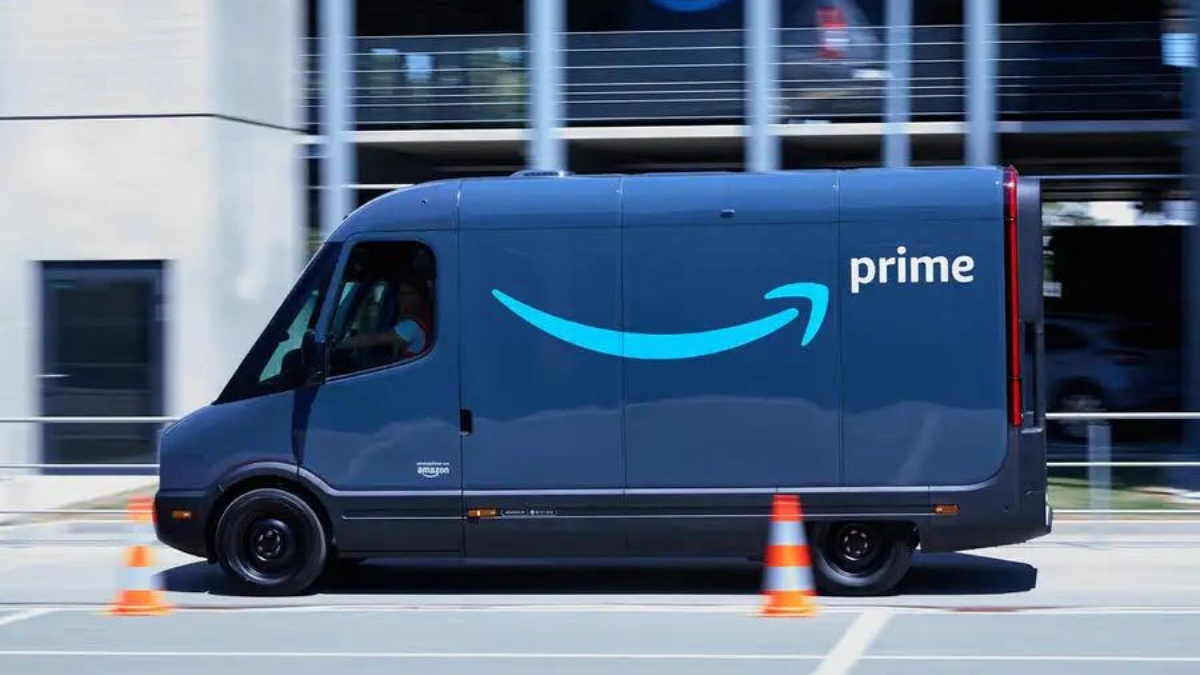A dynamic photograph captures an Amazon Prime delivery truck in motion on what appears to be a business street. The truck stands out in sharp focus amid a blurred background, suggesting its movement at the time of capture. Its signature blue color is highlighted by the prominent Amazon Prime logo on its side, featuring an upward-curving arrow resembling a smiley face, with the word "Prime" in clean, white text above it. In the driver's seat, a driver is visible, wearing a white shirt and what might be an orange safety vest.

The street scene includes orange and white striped construction cones; one is directly in front of the truck and another positioned near its back wheel. The backdrop features a parking garage with two visible levels, where several cars are parked. Near the front of the truck, a door leading to the parking structure can be seen, suggesting it provides access for vehicles. The setting and elements contribute to a bustling, urban atmosphere.